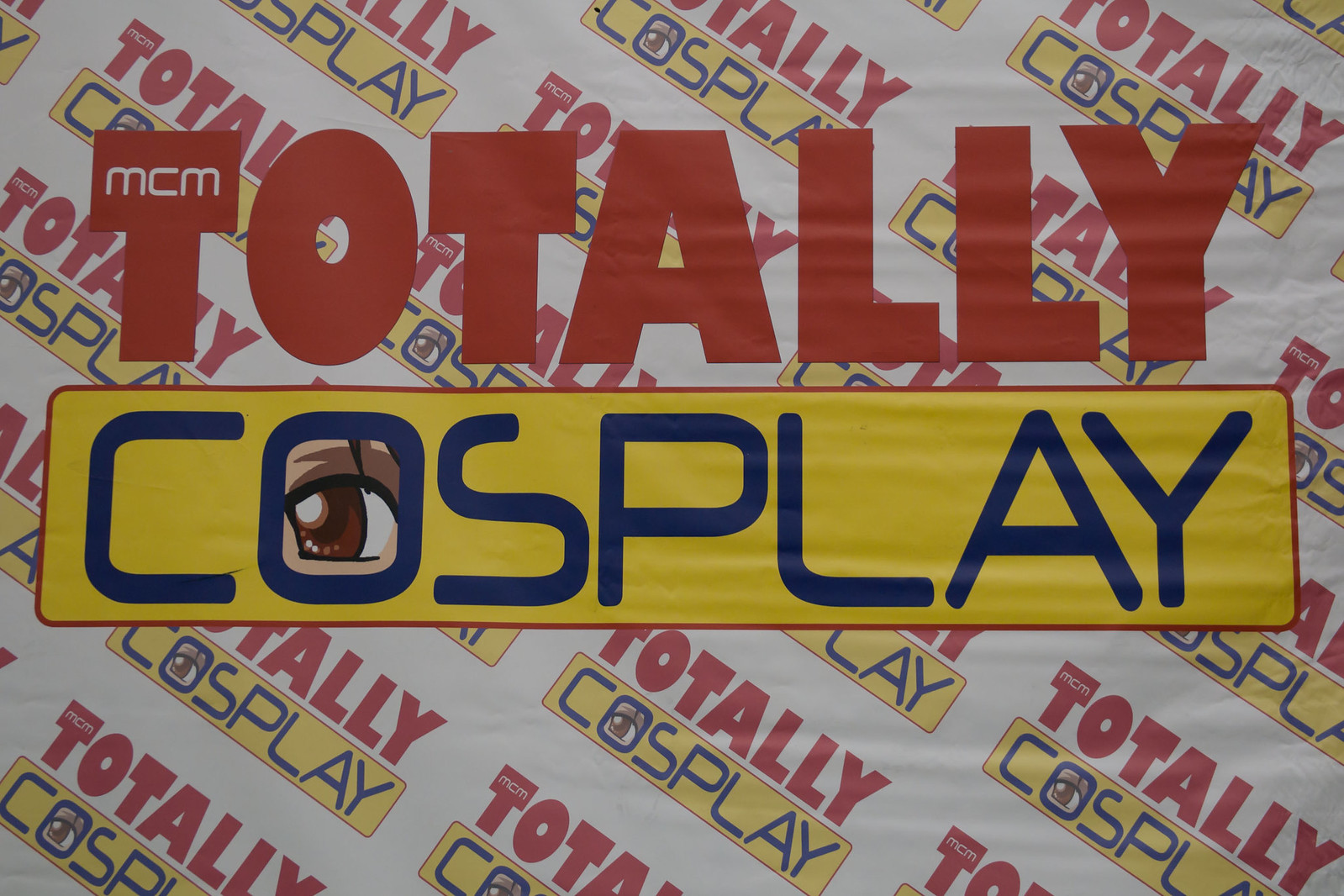The image showcases a wide, rectangular sign set against a white background patterned with repeated logos. The sign appears to be made of paper, with a noticeable crinkle in the top right corner. These logos are placed diagonally, slanting down to the right, and consist of two main parts aligned one above the other.

At the top, bold red capital letters spell out "TOTALLY," with the letters filled out and large. In the "T" of "TOTALLY," the initials "MCM" are inscribed in white letters. Beneath "TOTALLY," there is a yellow rectangle with a red border, containing the word "COSPLAY" in bright, dark blue capital letters. The "O" in "COSPLAY" features a brown, cartoonish eye on white skin, adding a quirky detail to the design.

The background is filled with a repeating pattern of the same logo—"TOTALLY COSPLAY"—scaled down and arranged diagonally to fill the space, creating a cohesive and branded appearance.